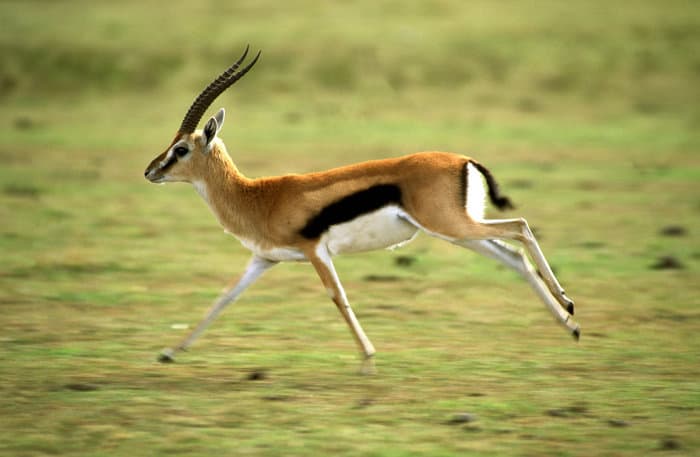The photograph captures a young gazelle in mid-run on a green, grassy area. The grass is short in the foreground but seems slightly longer and blurrier in the background, emphasizing the motion of the image. The gazelle is seen from the left side, with all four legs airborne, the front two just about to strike the ground. Its prominent black horns extend elegantly from its head, accompanied by two white ears. The gazelle's face features a distinctive white stripe from brow to nose, contrasted by a black line near its black eye. The upper half of its body is predominantly brown, with a striking black stripe running along its flank, and a pure white underbelly that extends to its rear. It also has a black tail and black hooves. The background is out of focus, further highlighting the gazelle's speed and motion, while the animal looks straight ahead, seemingly aware of being photographed.